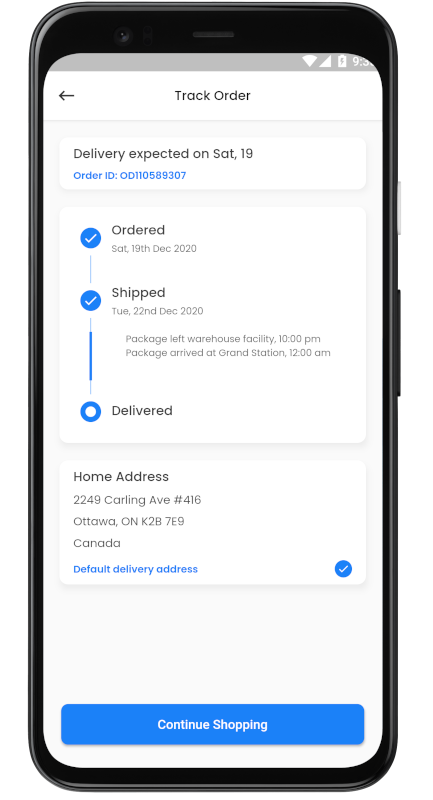**Detailed Caption:**

The image depicts a smartphone screen displaying the "Track Order" page of a delivery app. The background of the screen is predominantly black, while the top section has a lighter, white and grayish hue, with a small gray strip at the very top. The "Track Order" heading is prominently visible with a left-pointing arrow beside it. Below this heading, the text "Delivery expected on Saturday 19" is displayed, indicating the scheduled arrival date. Further down, in blue text, the order ID "OD 110589307" is shown.

Beneath the order ID, a rectangular section illustrates the order's progression via a tracking timeline. The first step is marked with a blue checkmark labeled "Ordered." A blue line extends down to the next step "Shipped," which is also marked with a blue checkmark. Another thin blue line continues downward to the final step, "Delivered," which is encircled in blue but remains unchecked, signifying that the order has not yet been delivered.

Continuing downward, another rectangular section displays the delivery address: "2249 Carling Avenue, Apartment 416, Ottawa, Ontario K2A 7S9, Canada." At the bottom of the screen, a bar with the text "Continue Shopping" provides an option for further shopping, suggesting it is clickable.